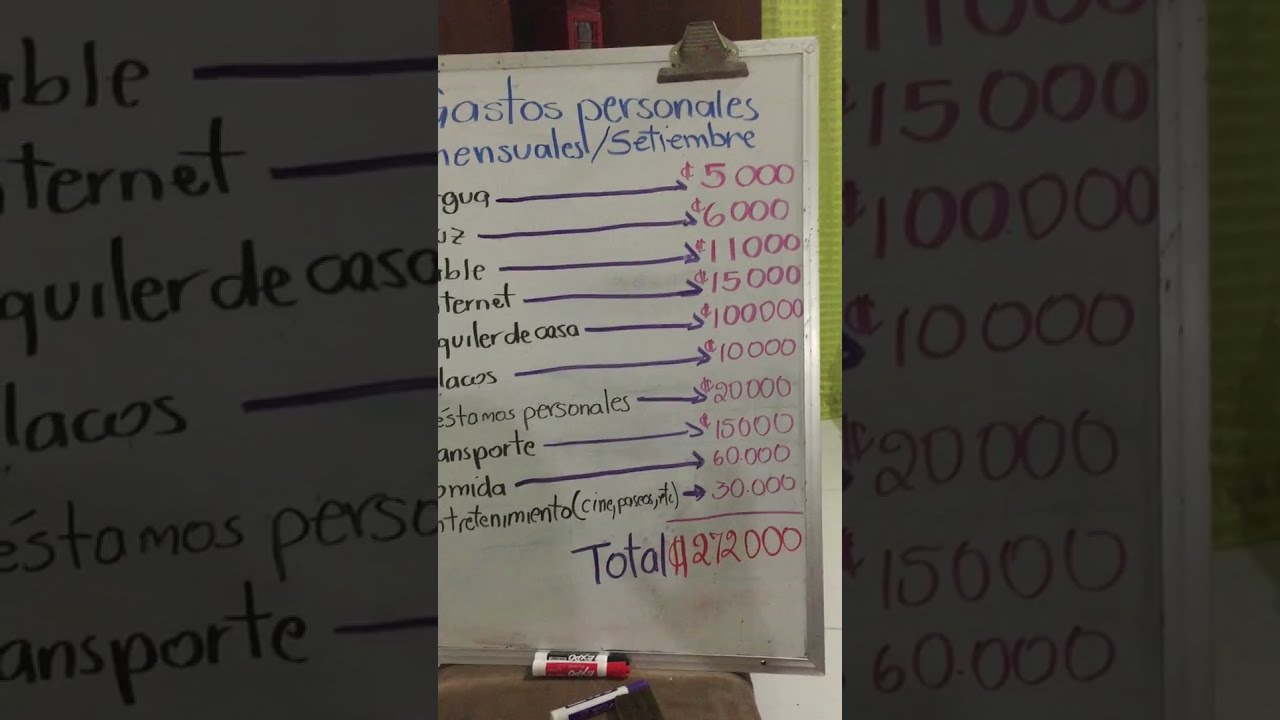The image is a horizontally aligned rectangular picture with thick black borders on both sides, framing a white background that appears to be a whiteboard rather than a sheet of paper. The whiteboard displays a detailed budget breakdown with the heading "Gastos Personales Mensuales Septiembre," written in blue. Below the heading, there are various items listed, though their names are partially obscured by the left black border. Each item has an associated number, presented in thousands, with figures written in red ink. These numbers are as follows: 5,000, 6,000, 11,000, 15,000, 100,000, 10,000, 20,000, 15,000, 60,000, and 30,000. There is a noticeable silver strip on the right side of the board, reinforcing that it is a whiteboard. A blue line totals these amounts, and the total sum of 272,000 is prominently written, the text "total" in blue and the amount in red. The currency symbol resembles a circle or a C with two lines through it, possibly indicating pesos or a similar currency.